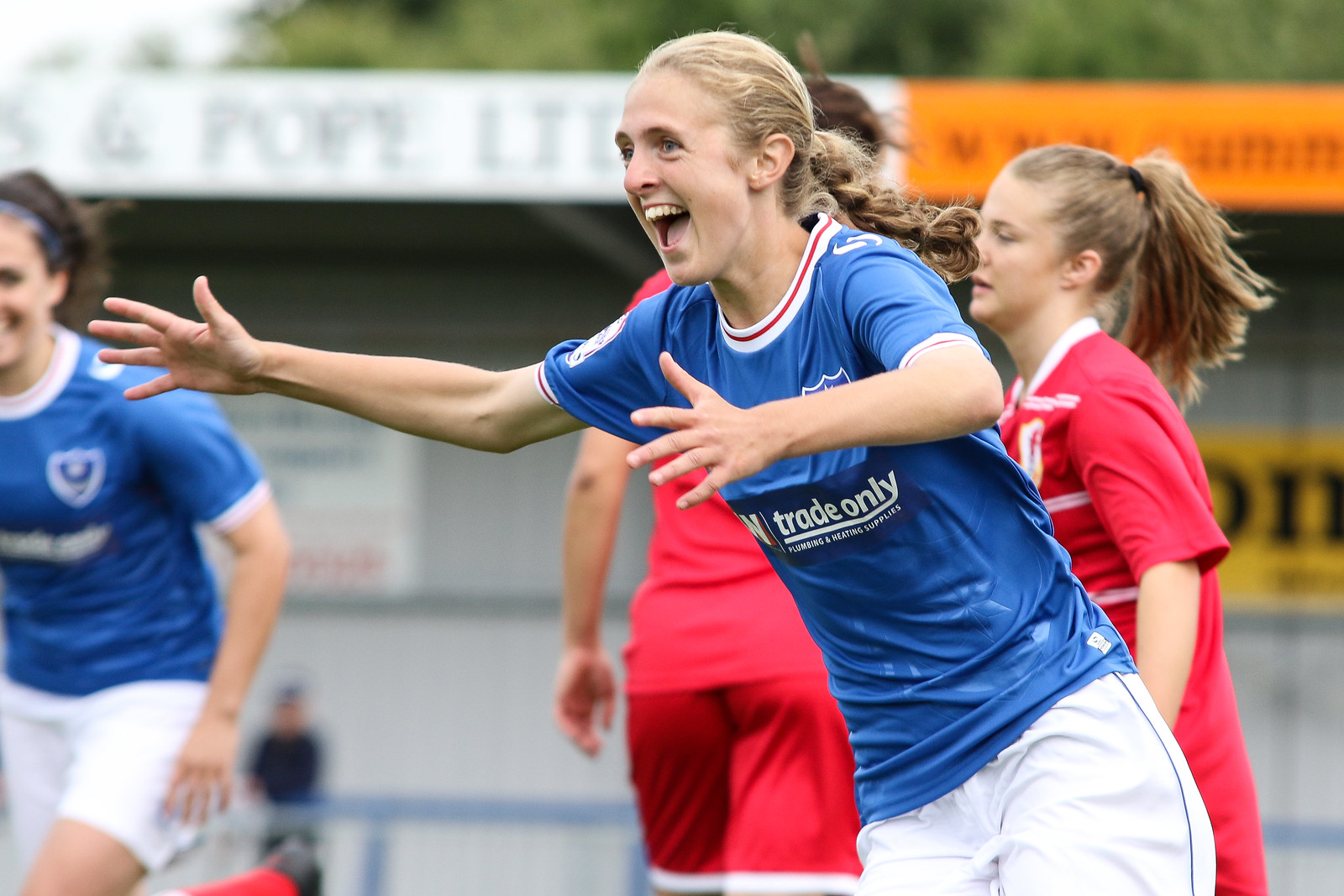The photograph captures a jubilant moment at a women's soccer game. Dominating the center of the image is a woman exuding happiness with her arms spread wide, her mouth open in an ecstatic expression, almost as if she’s ready to embrace someone. She is wearing a blue jersey with the words "Trade Only" emblazoned in white on the front, paired with white shorts. The jersey has a white neckline and white short sleeves with a red line running through it, revealing her arms up to her elbows. Her blonde hair is pulled back in a ponytail.

To the left, slightly blurry and in the background, another player can be seen in the same blue jersey, smiling at the central figure. Her brunette hair is distinguishable even through the blur. 

In stark contrast, positioned behind the jubilant woman, are two players in red jerseys and red shorts looking visibly tired and possibly defeated. One of these players has her back turned, while the other shows only half of her face. 

The backdrop features a mix of elements including a blurry building with orange accents and some unreadable writing, white stands or a wall, and greenery from nearby trees, suggesting the presence of a stadium setting with a hint of a concession stand or dugout area topped by a white awning.